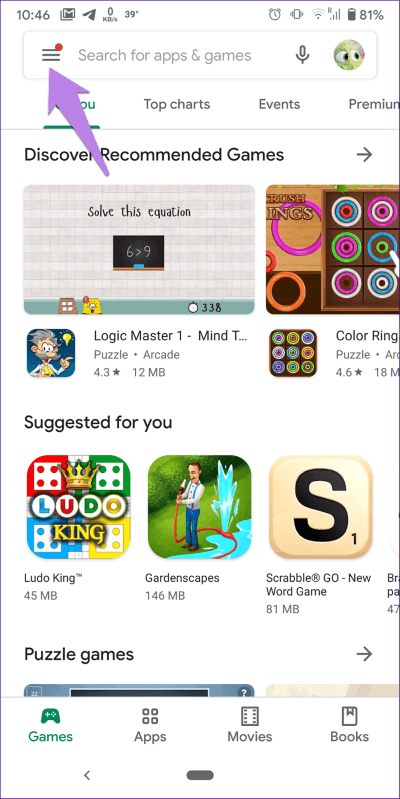The image features an iPhone screen displaying a snapshot of an app interface. The battery life is indicated at 81%, and the signal strength appears weak. The time shown is 10:46. At the top of the screen, there is a search bar with three horizontal lines on the left, each marked with a red circle on the upper right. A purple arrow points to these lines. To the right, there is an image of a green character next to a microphone icon.

Beneath the search bar, the headings "Top Charts," "Events," and "Premium" are visible, and there is a "For You" section below the purple arrow. A section labeled "Discover Recommended Games" follows, accompanied by an arrow pointing to the right.

Within this section, there are two game previews resembling the size of credit cards. The first game, "Logic Master," displays the message "Solve this equation: 6 > 9" and is categorized under puzzle and arcade games. The second game, "Color Rings," showcases colored rings.

Below these previews, there is a "Suggested" section with boxed recommendations for the games "Ludo King," "Gardenscapes," and "Scrabble." The bottom part of the screen hints at the category "Puzzle Games," though this is partially cut off. Additionally, there are icons for various categories, including games, apps, movies, and books, at the bottom of the screen.